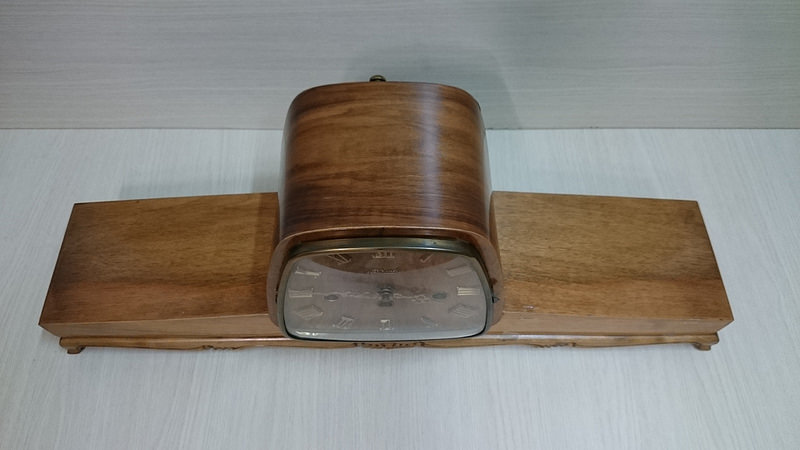This is a close-up photo of a detailed wooden clock, showcasing its intricate craftsmanship. The clock is made from light-stained wood and features an elegant and finely polished finish. The clock face is mounted on a cylindrical wooden base, which is flanked by two rectangular wooden blocks on either side, resembling wings. This distinctive design element adds a unique flair to the timepiece. The entire structure is supported by a brass platform, providing both stability and a touch of sophistication.

The clock face itself is brown, adorned with gold Roman numerals that stand out against the wooden backdrop. The hands of the clock are also gold, designed with ornate detailing that adds to the clock’s vintage charm. The clock is resting on a white, wood-grain painted table, matching the background, thus creating a harmonious setting. The polished glass covering the clock face reflects light, adding dimension to the photograph, while subtle shadows are cast behind the clock, enhancing its depth and presence in the image.